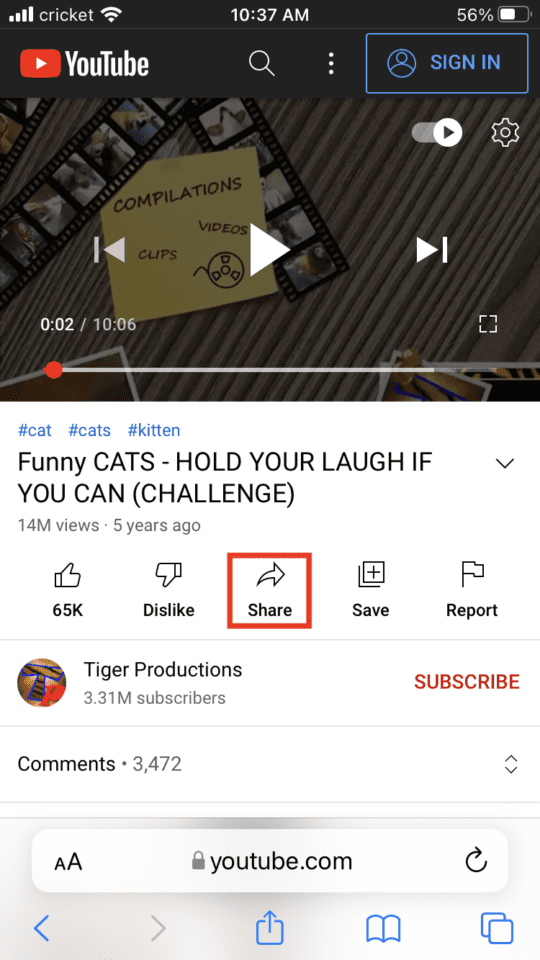In the screenshot, we see a YouTube video page with various interface elements. The top-left corner displays the network signal bar at full strength (3 out of 3 bars) from the provider Cricut's Wi-Fi. Centrally positioned at the top is the time, showing 10:37 AM, while on the top-right, the battery icon indicates a 56% charge.

The YouTube video at the center of the image has the title "Funny Cats Who Would You Love If You Can Challenge." The video is 10 minutes and 6 seconds long and was posted 5 years ago. It has garnered 14 million views and received 65,000 likes. The share button in the video interface is highlighted in red for easy visibility. The content is from the channel "Tiger Productions," which boasts 3.31 million subscribers. Additionally, there are 3,472 comments on the video.